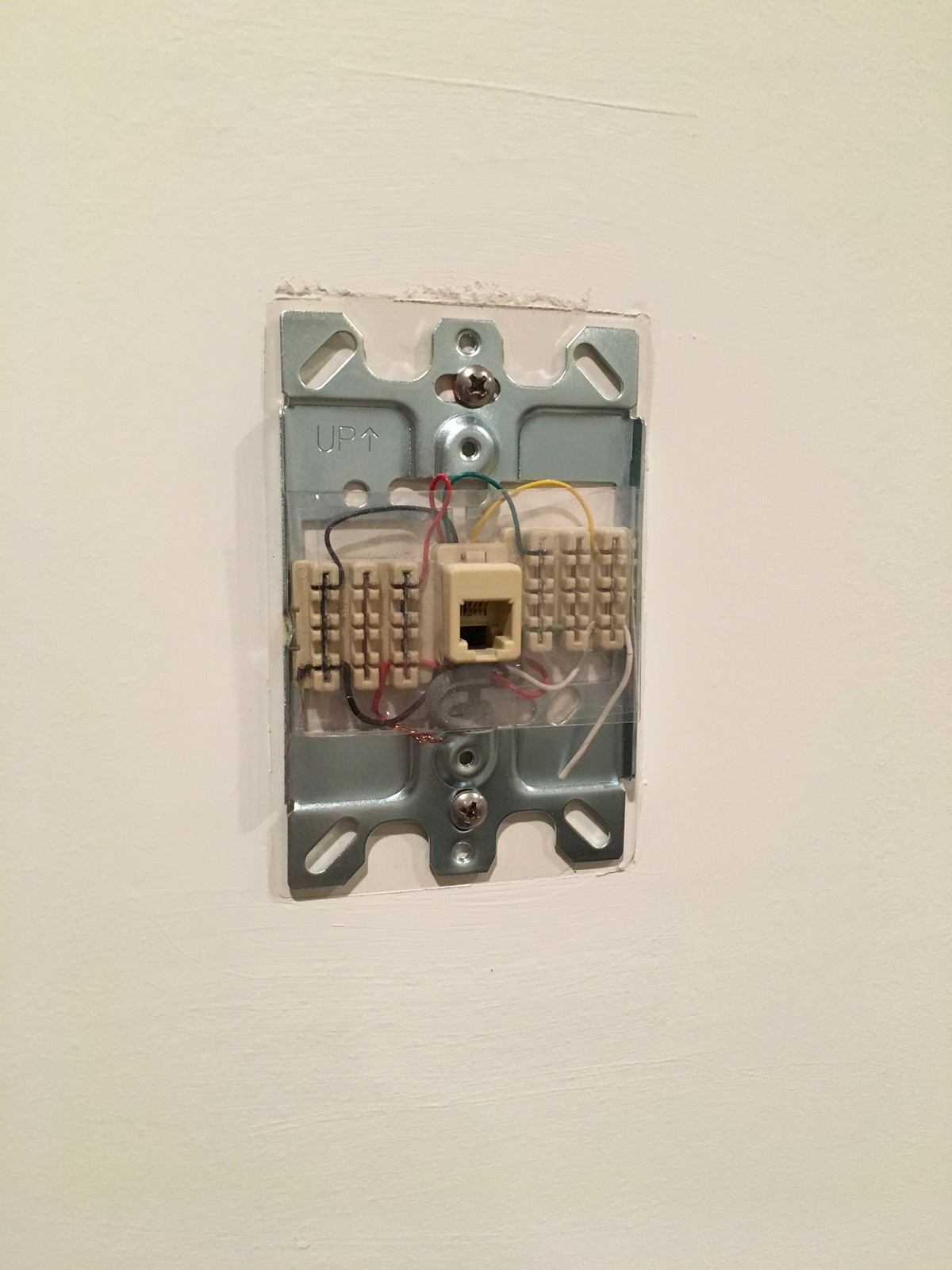The image showcases an electrical control panel mounted on a plain, flat white wall, which displays visible brush strokes from painting. The panel, framed in metal, features an engraving of an upward arrow labeled "UP," ensuring correct installation. The metal frame, dotted with various screws, suggests it is secure. Surrounding the frame is a noticeable line, possibly indicating where a cover, now removed, once protected the components within. This removal reveals the edges where the wall has been painted over or around the panel, resulting in a slight elevation from layers of paint.

Inside, the panel contains a central plastic component, now markedly yellowed with age. The discoloration implies it has never been exposed to direct sunlight but has aged naturally over time. Various colored wires—black, red, green, yellow, and white—are interwoven through the central component, hinting at the complexity and functionality typical of control panels. This detailed exposure invites a deeper curiosity about the panel’s purpose and history.